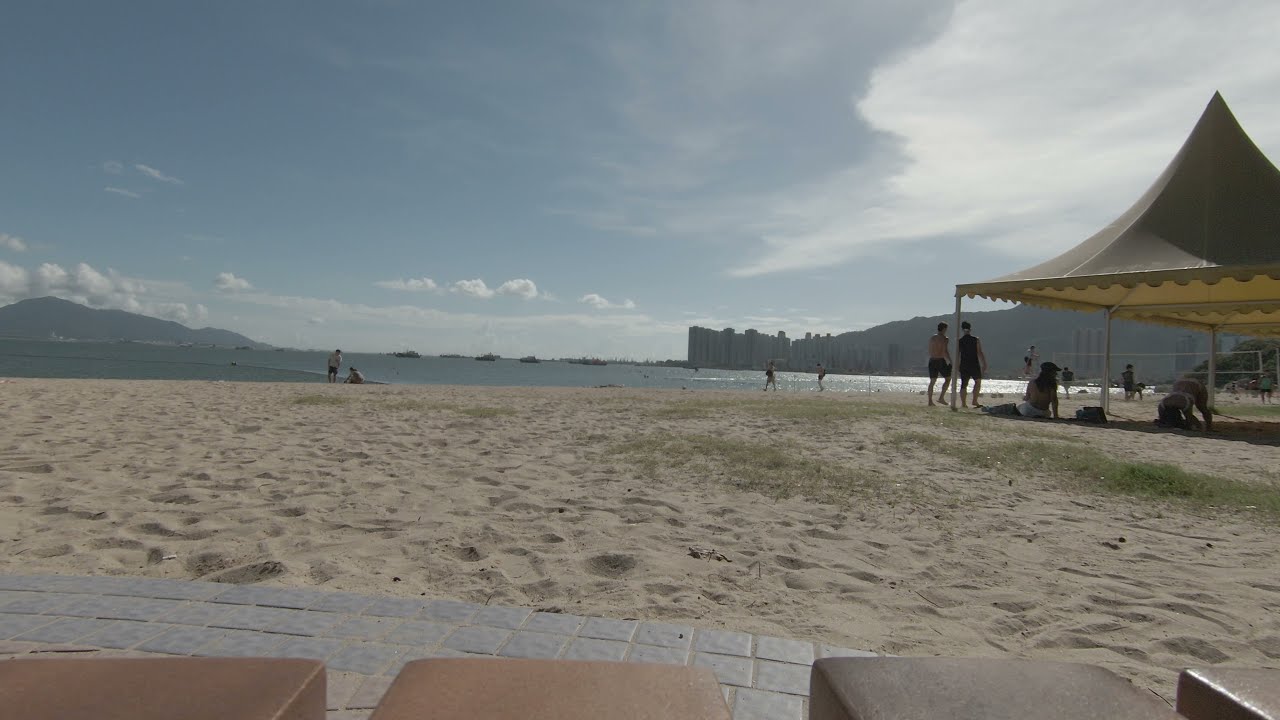This horizontal, rectangular image captures a busy beach scene, now empty, yet bustling with evidence of past activity, such as numerous footprints etched into the expansive sandy area that stretches halfway up the photograph. In the foreground, a stone walkway and some pillars suggest a patio or terrace area from where the picture was taken, possibly from a chair. To the right, there is a large, open canopy tent likely meant for picnicking, though devoid of tables. The beach was recently active, with people seen strolling, some under the canopy, others in the sand, and a few in the water. The background reveals a cloudy, overcast sky indicating it might be late in the day. Beyond the beach, calm waters sparkle subtly under the dimming sunlight. Distant mountainous landforms jut out on either side of the beach, offering a semi-enclosed natural frame. Further out, ships or boats are visible against the horizon. On one side, the mountains exhibit a unique, structured appearance reminiscent of rectangular prisms or monumental pillars, adding an intriguing geometric element to the otherwise organic landscape. Skyscrapers from an adjacent city can be seen faintly through the haze, melding the boundaries of nature and human development.